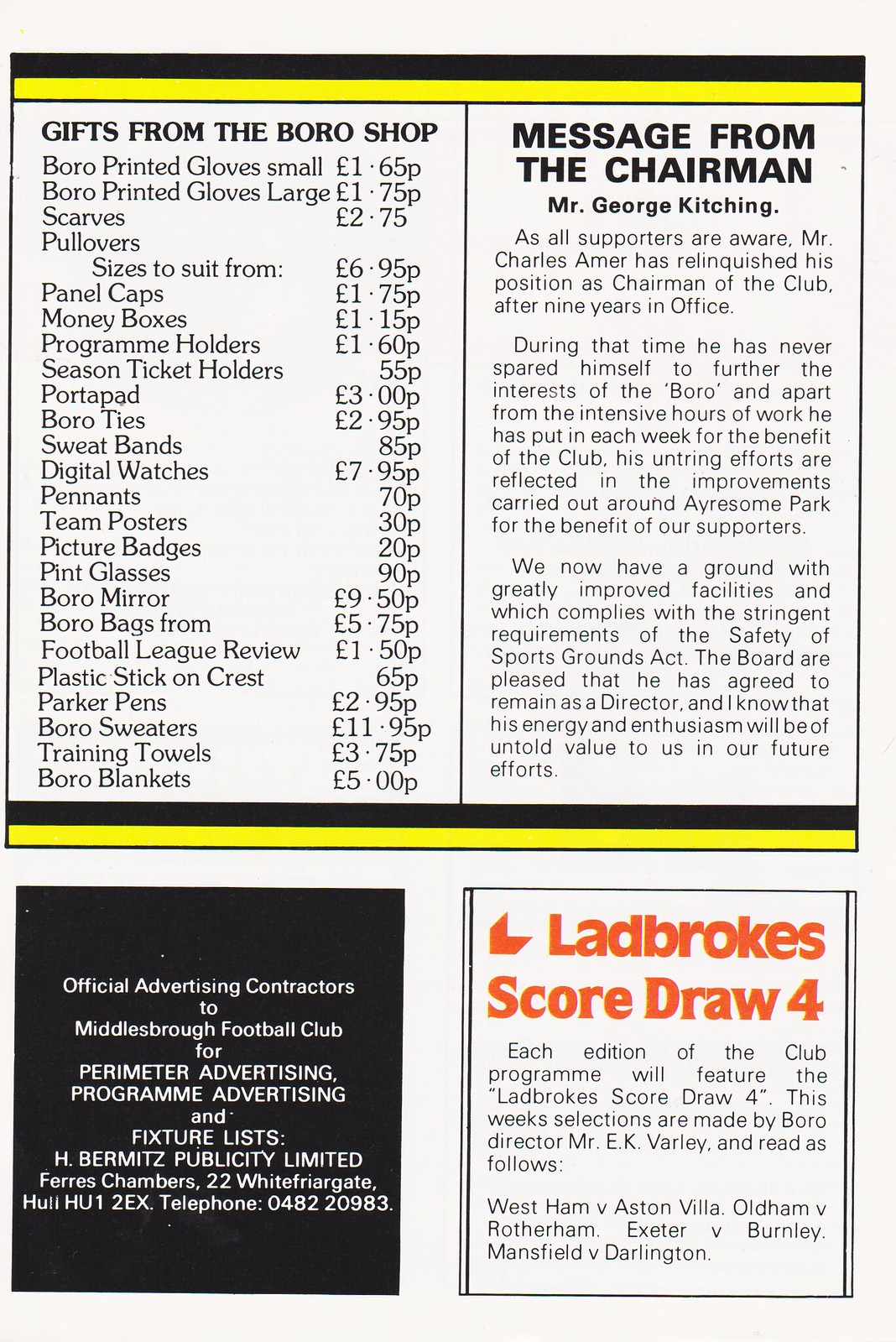This is a page from a game day program for Middlesbrough Football Club, divided into several sections. The top half is split into two columns. The left column, titled "Gifts from the Borough Shop," lists various items for sale along with their prices, including printed gloves (small for 1 euro 65p, large for 1 euro 75p), scarves, pullovers, panel caps, money boxes, program holders, season ticket holders, Port-A-Pad, Borough ties, and more. 

The right column features an article titled "Message from the Chairman, Mr. George Kitching," which details the retirement of Mr. Charles Amor from his position as chairman after nine years of dedicated service. It highlights his substantial contributions to the club, including the intensive hours of work and improvements made to Iresome Park to meet the Safety of the Sports Grounds Act requirements. Though stepping down as chairman, Mr. Amor will continue to serve as a director, bringing his energy and enthusiasm to future efforts.

The bottom of the page is divided into two parts. The bottom left contains a black square with white text that reads, "Official Advertising Contractors to Middlesbrough Football Club for Perimeter Advertising, Program Advertising, and Fixture Lists." The bottom right features an advertisement for "Ladbrokes Score Draw," mentioning that each edition of the club program will include selections made by Borough Director, Mr. E.K. Varley, with this week's games being Westham v. Aston Villa, Oldham v. Rotherham, Exeter v. Burnley, and Mansfield v. Darlington. The page is visually framed with black and yellow borders.